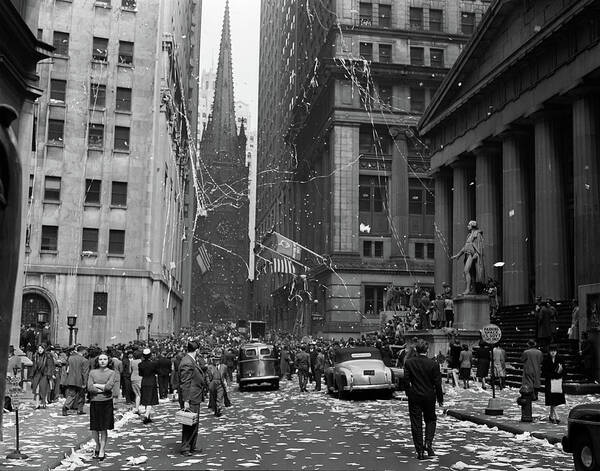This black-and-white photograph captures the lively scene of a ticker tape parade, likely in New York City. Streamers and ticker tape cascade through the air, creating a festive atmosphere. The street is densely populated with hundreds of people dressed in 1960s-era clothing; women are in dresses, sweaters, and heels, while men are mostly in suits. The ground is littered with papers and confetti, evidence of the recent celebration.

To the left of the street, a stately building with Corinthian columns stands prominently. On the right, a notable stone statue of a man holding a sword is perched high above the bustling crowd below. Further along the street, two towering skyscrapers frame the background, directing the eye toward a grand cathedral spire visible between them. American flags hang from several buildings, adding to the patriotic ambiance. Vintage cars from the 1950s and 60s, with their characteristic rounded fenders and all-metal bodies, line the street, completing the nostalgic scene.